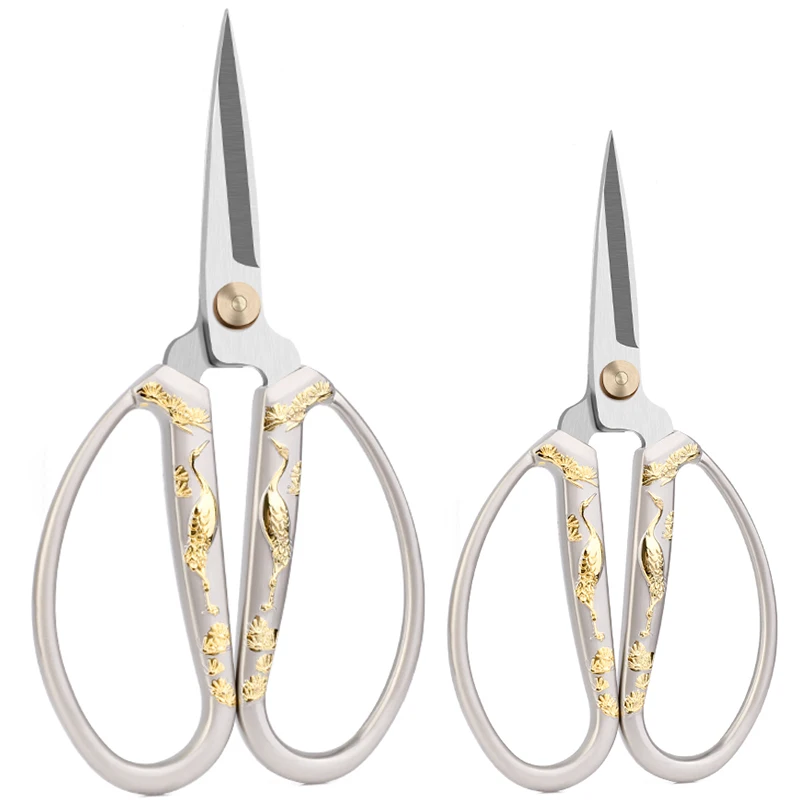The image showcases two pairs of ornate embroidery scissors displayed on a white background. These scissors are distinctively adorned with intricate gold filigree in the shape of cranes, positioned with their heads facing inward towards the blades. Each crane's elegant form continues down the handles, with one leg lifted and the other crossed, evoking a natural stance. Surrounding the cranes are delicate engravings that resemble lily pads and marsh plants. The handles of the scissors are large and oval, featuring a light platinum color with gold artwork inside. The short blades are silver-toned, and the pivot points, which are a slightly darker copper or bronze color, hold the scissors together. The larger pair is positioned on the left, complementing the smaller pair on the right, making it an ideal product showcase image for potential purchasers.